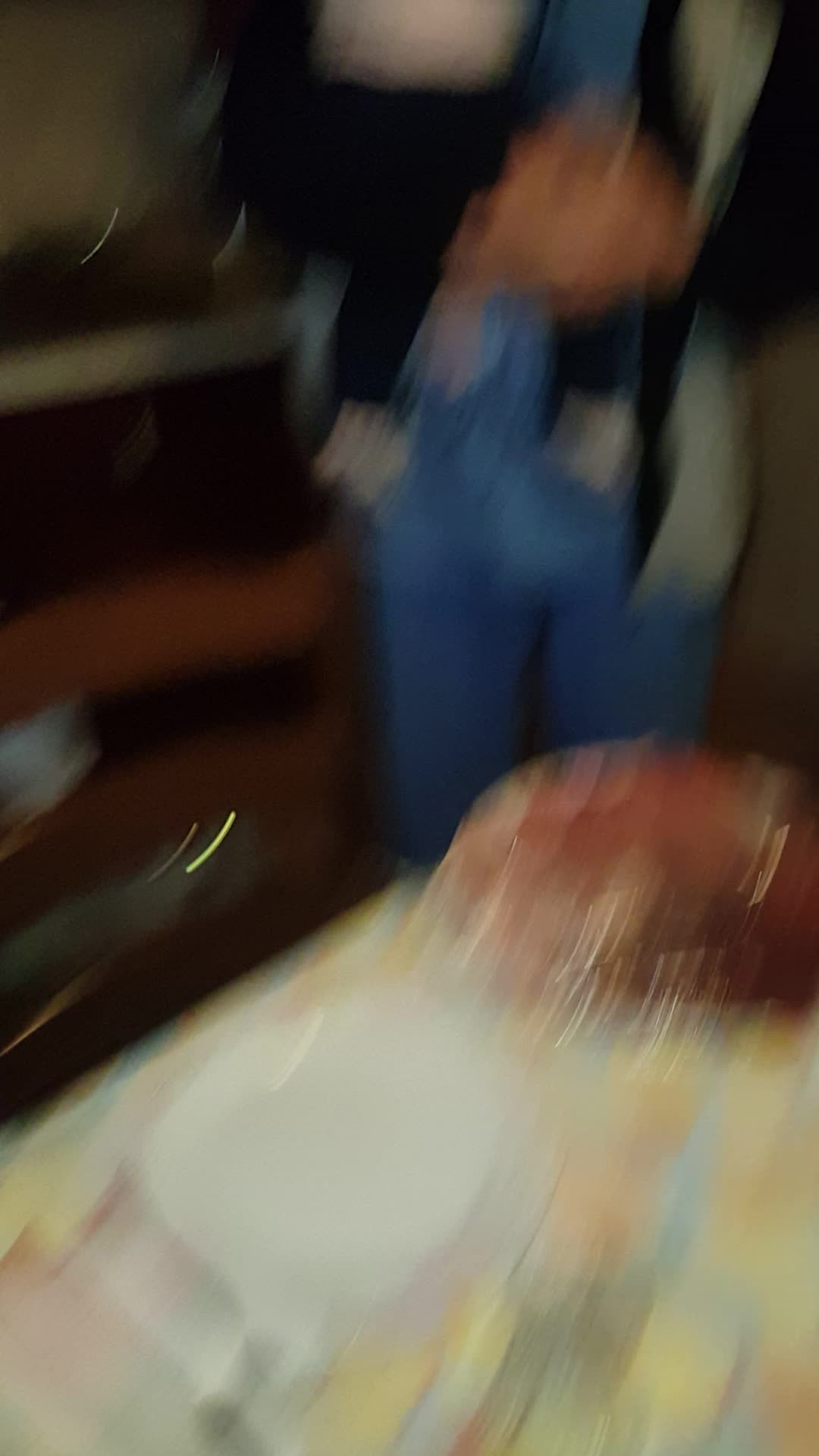In this extremely blurry photograph, likely taken in motion, the central subject appears to be a person with brown hair and bangs, wearing a blue shirt and jeans. The person seems to be holding something indistinct in their hands—potentially a small baby or stuffed toy, as suggested by the sight of small, dangling arms, although the "head" area is too blurry to confirm. In the foreground, there is a table with a yellow floral cloth, bearing a plate of food, possibly a cake or pie with a red topping like cherries or strawberries. The background is dark with some gray and tan shades, indicating they might be indoors, with green light flashes adding to the overall haze of the image.